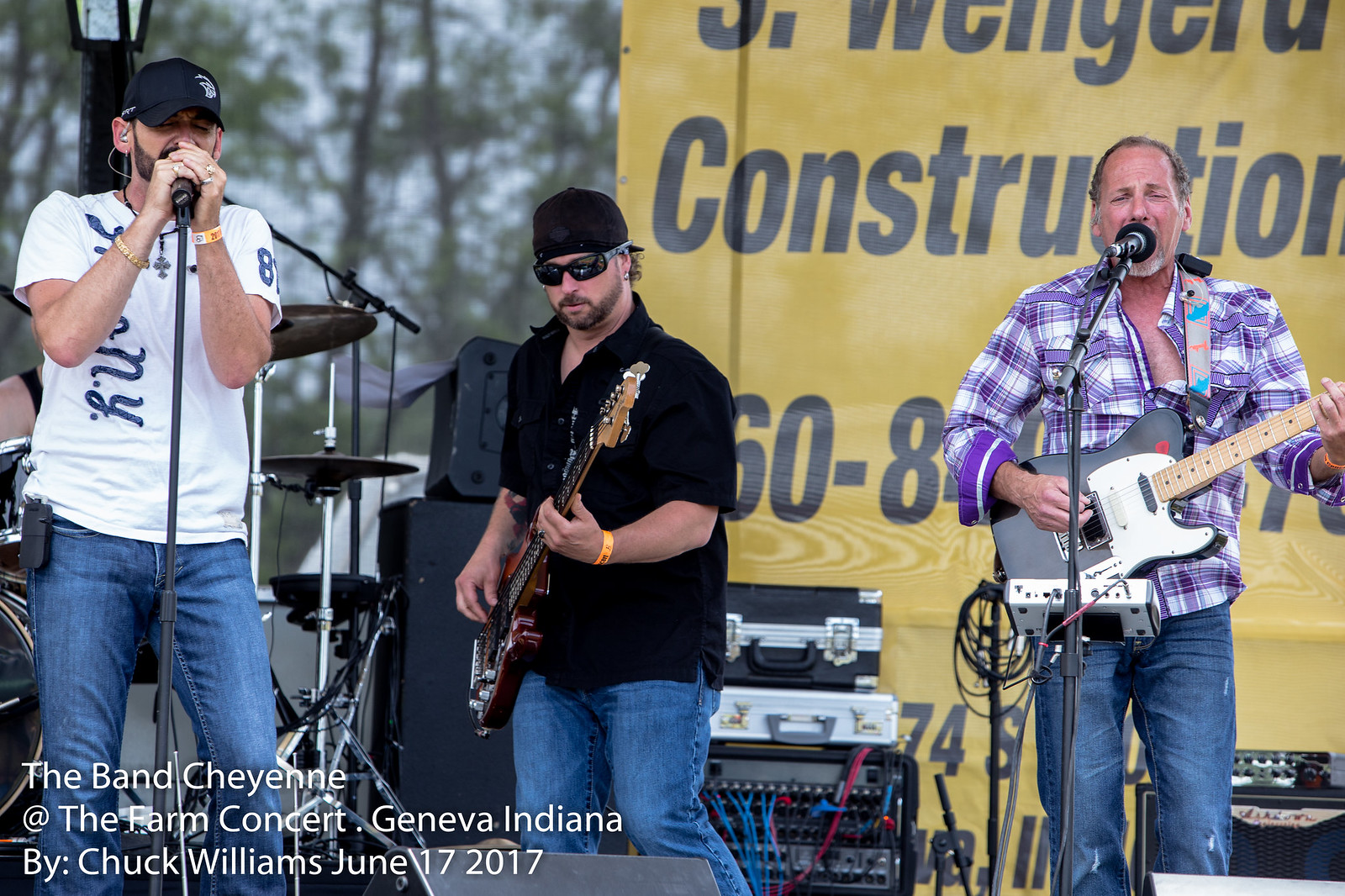The image captures a lively performance by the band Cheyenne at the Farm Concert in Geneva, Indiana, held on June 17, 2017, and photographed by Chuck Williams. Three men are on stage: the man on the left is singing into a microphone, dressed in a black baseball cap, a white short-sleeved shirt, and blue jeans. He is notably the tallest of the three. The man in the middle, also singing, is the shortest and is playing a red and black guitar. He wears a black backwards baseball cap, sunglasses, a black short-sleeved shirt, and blue jeans. The man on the right, who has a light beard and thinning hair, is singing and playing a black and white electric guitar. He is clad in a white and purple striped shirt with blue jeans and stands in front of a microphone. Behind them, a big yellow sign with partially obscured black letters reads "CONSTRUCTION" and displays the numbers "60-8." The setup includes various musical instruments, such as a drum set, and trees are visible in the backdrop. The text in white at the bottom left of the image states, "The Band Cheyenne at the Farm Concert, Geneva, Indiana by Chuck Williams, June 17, 2017."